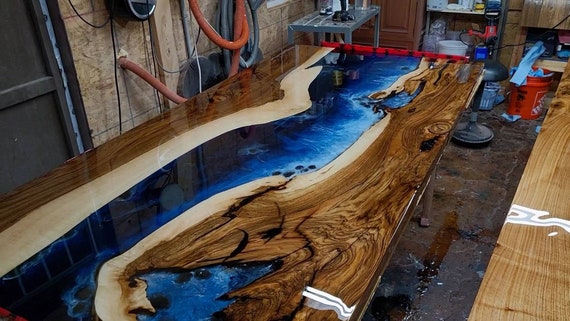This image captures an interior workshop, viewed from above, with a rich display of craftsmanship and tools organized in a well-lit room. The focus of the photograph is a highly glossed, beautifully oiled wood carving prominently featuring a river of blue that spans diagonally from the bottom left to the top right of the image, creating a stunning visual effect. The carving rests on a table with a backdrop of various shades of light to dark brown hues, enhancing the natural aesthetic of the workspace.

The room's floor is covered in wood, with a dark brown industrial carpet in the bottom right corner, wet with a splash of water. To the left of the carving, a wood-paneled wall with orange hoses is visible, contrasting with a large gray table behind the artwork in the upper left. This table supports several items, indicating active use. Against the back wall are shelves stocked with containers, tools, and machinery essential for the craft. 

An orange Home Depot pail is noticeably placed in the upper right corner, and a black stool stands beside the gray table, next to more wood boards arranged along the right side of the room. The overall scene is a harmonious blend of detailed craftsmanship and a well-equipped workshop environment, highlighting both the beauty of the wood carving and the practicality of the working space.